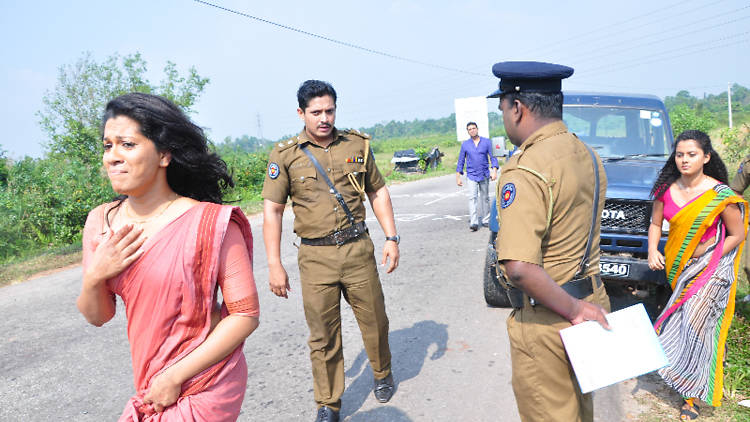This photograph appears to have been taken in a rural area of India, possibly in the outskirts away from a city, based on the dry grasslands, sparse trees, and power lines in the background. The scene is set on a sunny, hazy day, with several figures captured in the image. To the right, there's an older model blue Toyota truck, partially obscured by the people in the foreground.

Prominent in the foreground are two Indian women and two police officers. The officers are dressed in khaki uniforms with badges and crossbody utility belts; one of them wears a beret-like police hat. One officer appears to be facing the camera while the other stands with his back to it. One officer also seems to be escorting one of the women away from the vehicle. The women are dressed in traditional brightly colored saris. The woman in the pink sari seems particularly distressed, holding one hand to her chest and gripping her sari with the other as if she is about to cry or is already crying. She is moving away from the scene quickly, indicating her emotional turmoil.

The other woman is dressed in a multicolored sari with shades of pink, yellow, and blue, and appears to be following the first woman. A man dressed in business casual attire—light-colored jeans and a blue button-down shirt with rolled-up sleeves—walks toward the group from the background, looking curious or concerned about the situation.

The overall atmosphere suggests a tense moment, possibly involving the detainment of the two women by the officers. The expressions and body language indicate confusion, sadness, and distress.